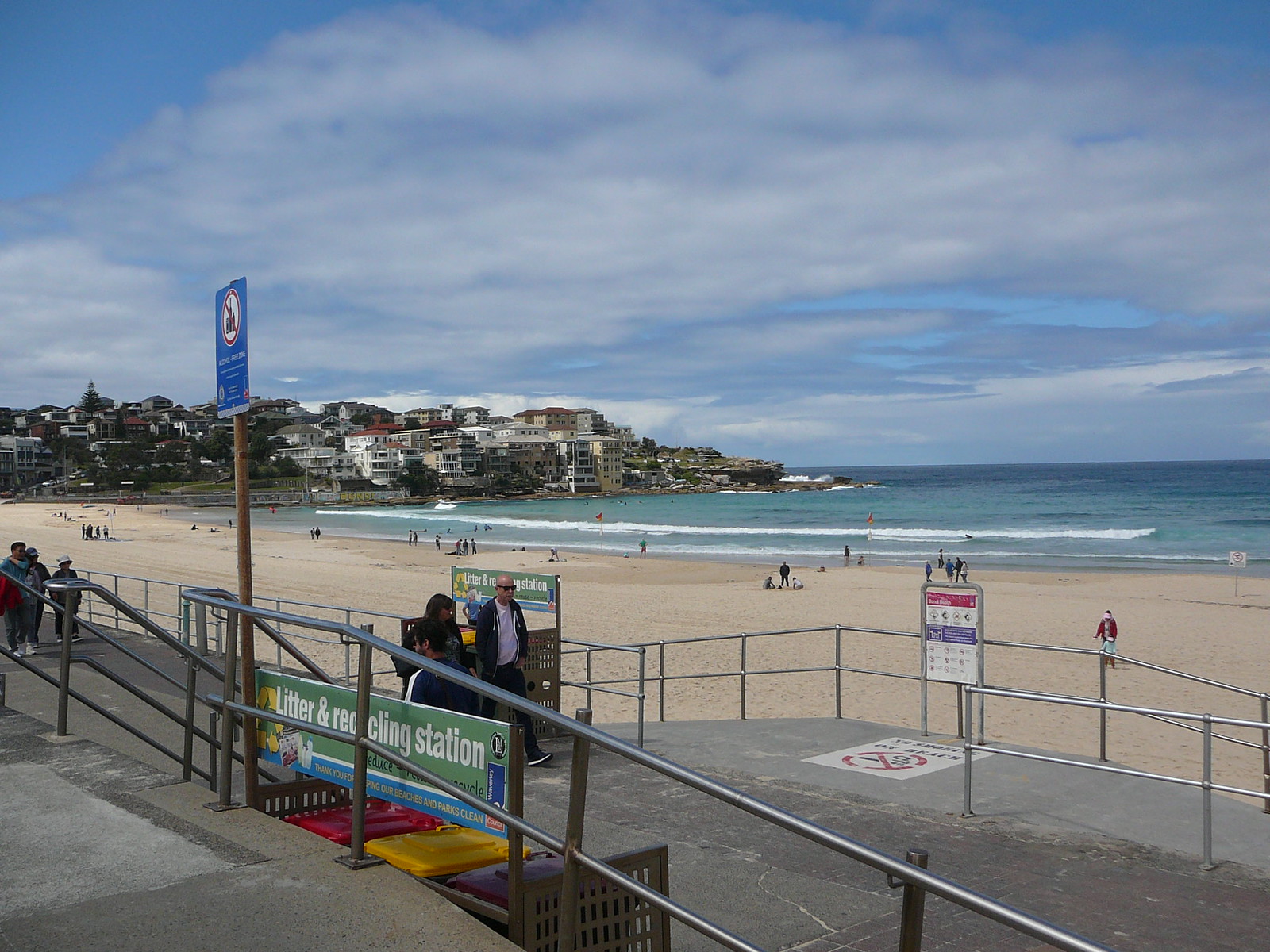The image captures a bustling beach scene on an overcast day, likely in an American coastal town, as suggested by the numerous signs and advertisements. In the foreground, a wide ramp with railings on both sides extends from the right side to the left, dotted with recycling stations featuring colorful lids in red, yellow, and purple. A couple of people, dressed in spring jackets and pants, are seen walking up the ramp, appearing to enjoy their day despite the cooler weather. The sandy beach stretches from right to left, meeting the ocean tide that is visibly coming in. Numerous people can be seen along the shoreline, either walking or sitting, although none are swimming, hinting at the chill in the air. In the background, an array of buildings and houses line the water's edge, suggesting a densely populated area. The sky above is a mix of clouds and clear patches, adding a tranquil ambiance to the coastal vista.